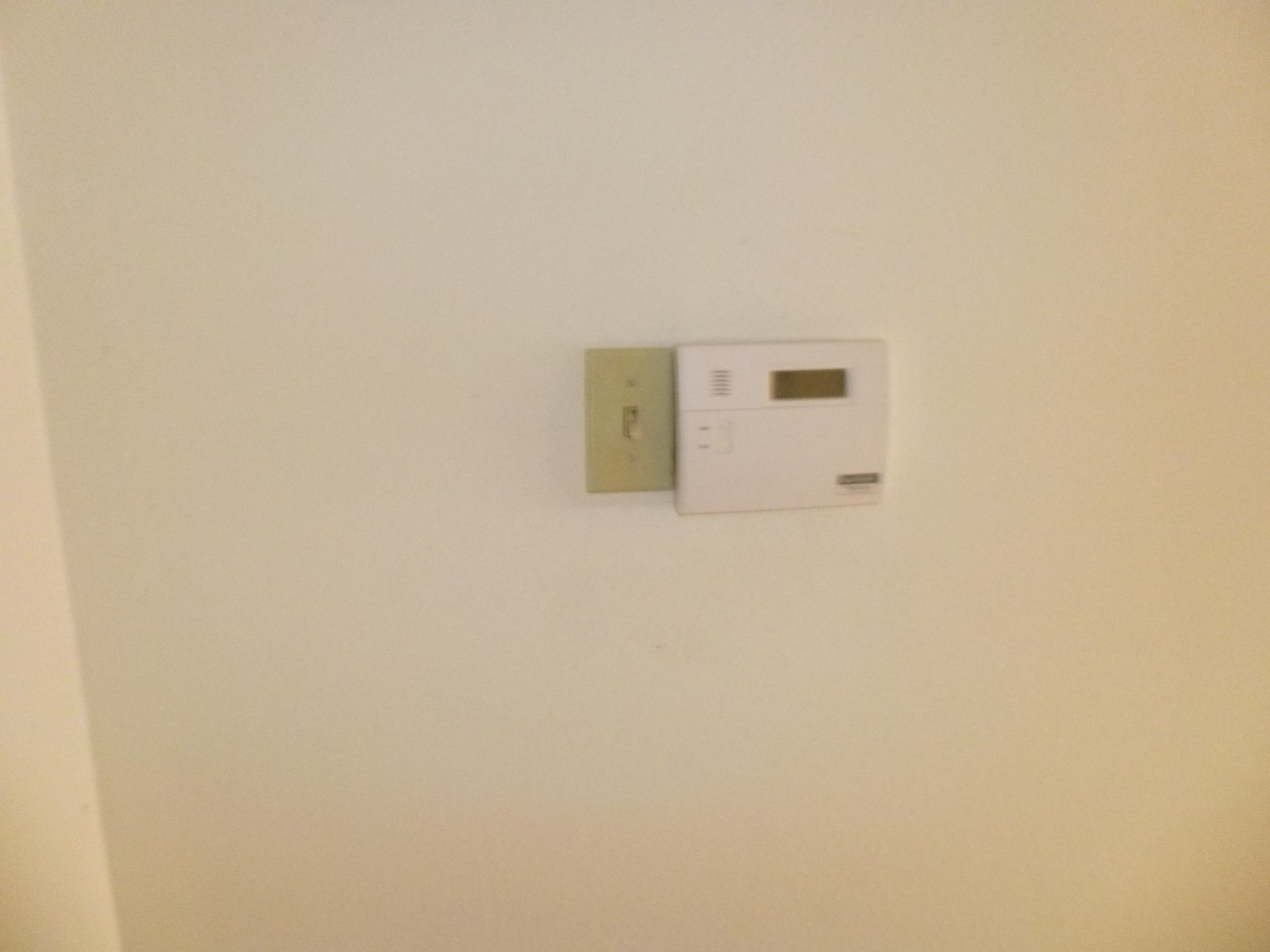A minimalist white wall features two distinct fixtures centrally positioned. The first, a brownish rectangular light switch with a noticeable black outline, is located roughly in the center of the image. This switch, oriented vertically, is flicked off to the right. Adjacent to the right of the light switch is a slightly larger device designed for controlling heating and air conditioning. It is a white box, about twice as wide as the light switch, and extends a bit lower. 

The temperature control device includes six small ventilation slits on the upper left side and a rectangular screen displaying the current temperature to the right of the slits. Just below, a faint horizontal line suggests a hinge or opening mechanism for accessing the interior of the device. In the bottom right corner of this device, a black banner with white, unreadable text is visible. The entire setup is against a subtly two-toned white backdrop, with the leftmost side appearing slightly whiter than the rest of the dingier white wall.